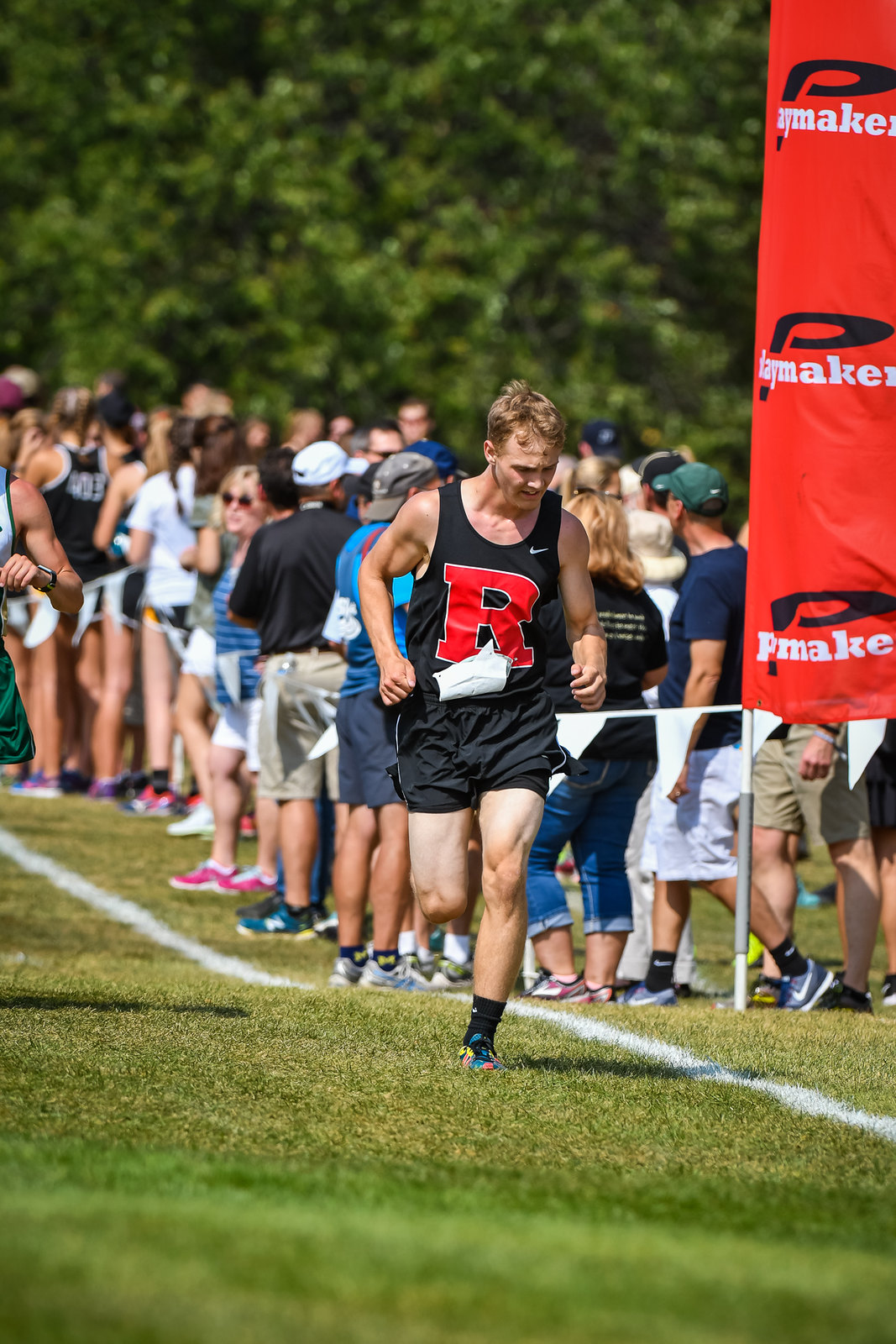In the image, a runner wearing a black, sleeveless Rutgers running outfit with a prominent red 'R' and a Nike swoosh is captured in motion on a short grass track. The runner, who appears to have a prosthetic leg, is seen likely holding it as he navigates the course, possibly hobbling on one foot, with his shorts and black socks adding to his athletic attire. A clearly marked white line runs alongside him, separating him from a decent-sized crowd of spectators who are watching attentively. On the far left, the arm of a second runner is partially visible, hinting at the presence of other competitors. In the background, there is green foliage towering above the crowd, and to the right, a flag bearing the Playmaker logo, possibly of the event sponsor, is prominently displayed.